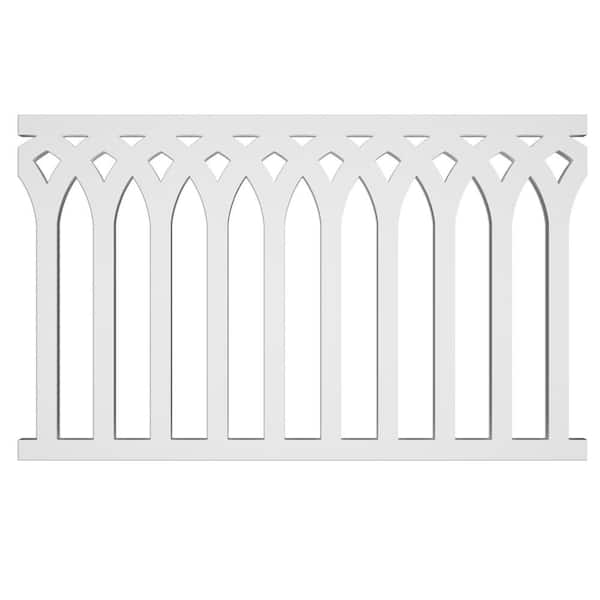The image depicts a single segment of a decorative white fence, set against a plain white background, giving no indication of scale. The fence itself features a repetitive pattern of curved gaps and overlapping arches, creating an intricate design. The top of the fence is adorned with small triangle and diamond-shaped cutouts, adding a creative touch to its otherwise plain appearance. Vertical lines accentuate the section, connecting to form a lattice-like design. This segment appears as if it could be one of multiple pieces that can be combined to form a continuous fence, potentially used to enhance a wall or garden area. The fence is presented front-on, without showing its thickness or any additional context.